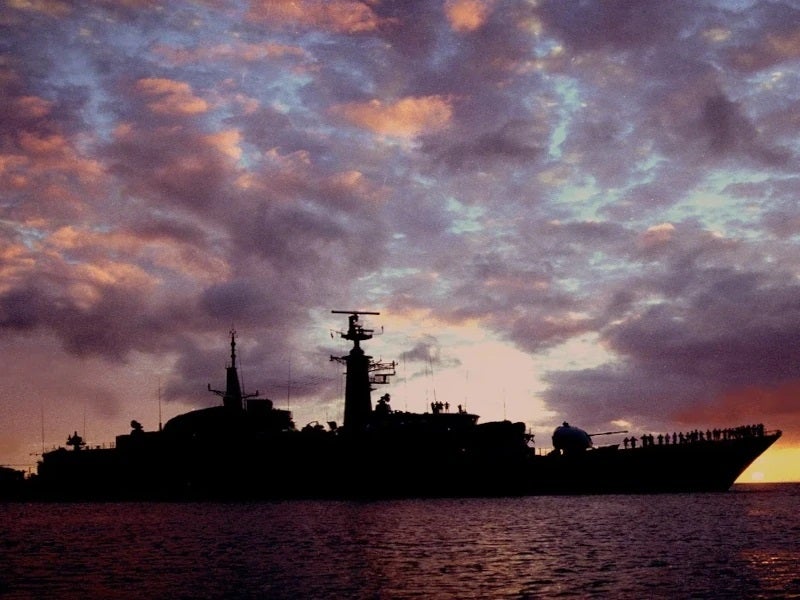This dramatic evening photograph captures a silhouetted Navy battleship navigating through the ocean. The vast vessel, shrouded in darkness due to the setting sun, reveals only its imposing shape against a backdrop of a gray, blue, and orange-tinted sky. Prominent features include a large tower at the front equipped with radar and multiple antennas. The bridge, positioned further aft, also sports antenna masts. On the bow, a distinct silhouette of a turret gun can be seen, adding to the ship's formidable appearance. Approximately 35 to 50 sailors are lined up along the bow’s railing, their shadows stark against the ship's dark outline. The tranquil yet powerful scene is complemented by the quiet, gray sea below the ship, hinting at the close of day with subtle hints of the sun in the lower right corner.